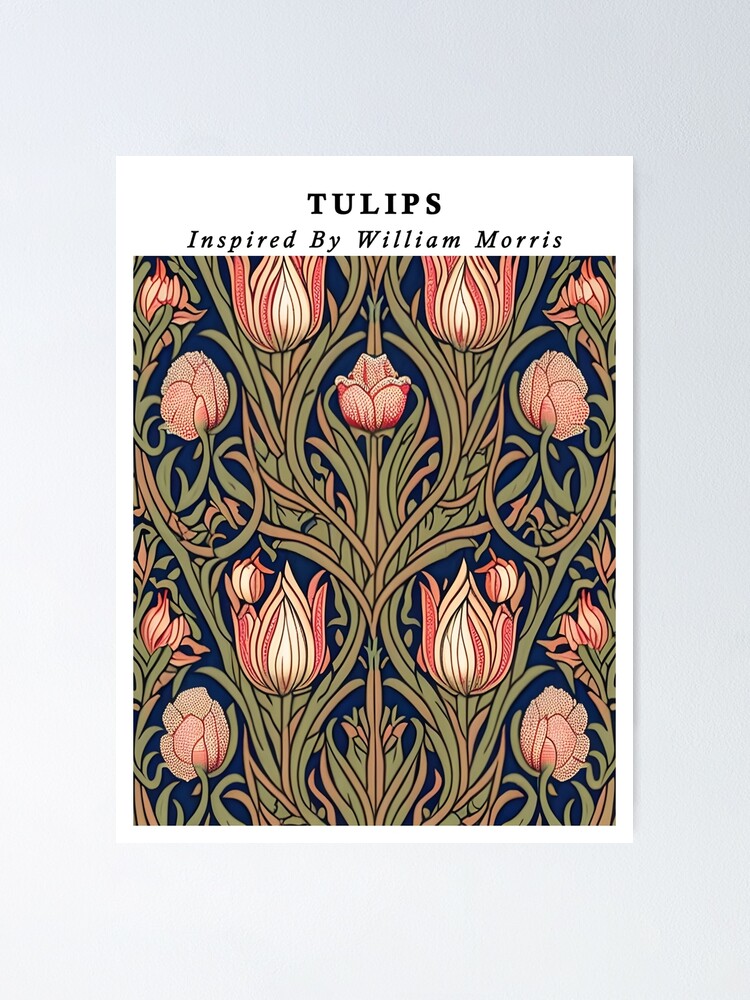The image is a detailed poster titled "Tulips Inspired by William Morris," capturing the essence of William Morris's Arts and Crafts style from England. This intricate design, reminiscent of traditional Morris wallpapers, features an ornate pattern dominated by lush green foliage intertwined with flowers. The flowers, although tulip-shaped, come in shades of white and pink, interspersed with additional floral elements such as roses. The blossoms are depicted in various stages of blooming, from buds to full blossoms. The entire arrangement, which contains approximately four tulips and five roses, is set against a deep, dark background, either black or very dark blue, enhancing the vivid colors of the foliage and flowers. The leaves and stems create a swirling, scroll-like effect in green and olive, complementing the salmon-colored leaves and heightening the overall intricate, geometric feel of the design.